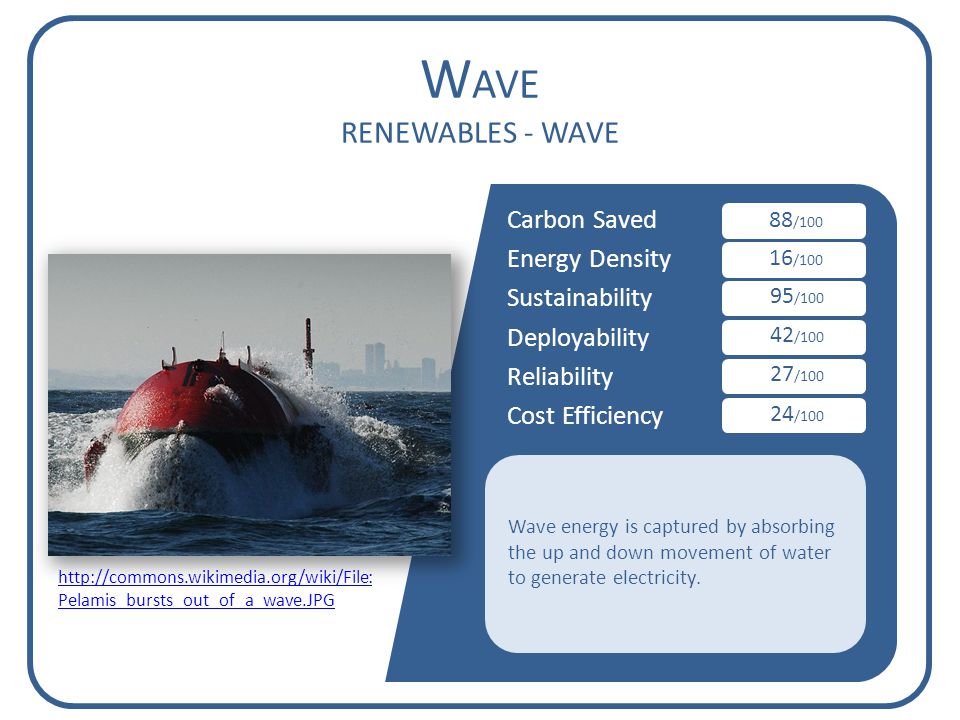The image prominently displays the word "WAVE" at the top in large font, followed by the sub-caption "Renewables Wave" in all capital letters but in a smaller font size. Below the titles, a list of environmental metrics is presented, detailing various aspects of wave energy:

- Carbon Saved: 88/100
- Energy Density: 16/100
- Sustainability: 95/100
- Deployability: 42/100
- Reliability: 27/100
- Cost: 24/100

Additionally, the caption explains that wave energy is harvested by harnessing the up-and-down movement of water to generate electricity. Featured beneath the primary photograph is a link: "http://commons.wikimedia.org/wiki/File:Palamas_bursts_out_of_a_wave.jpg." The image linked shows a red contraption emerging from the ocean, presumably an apparatus designed for wave energy capture.